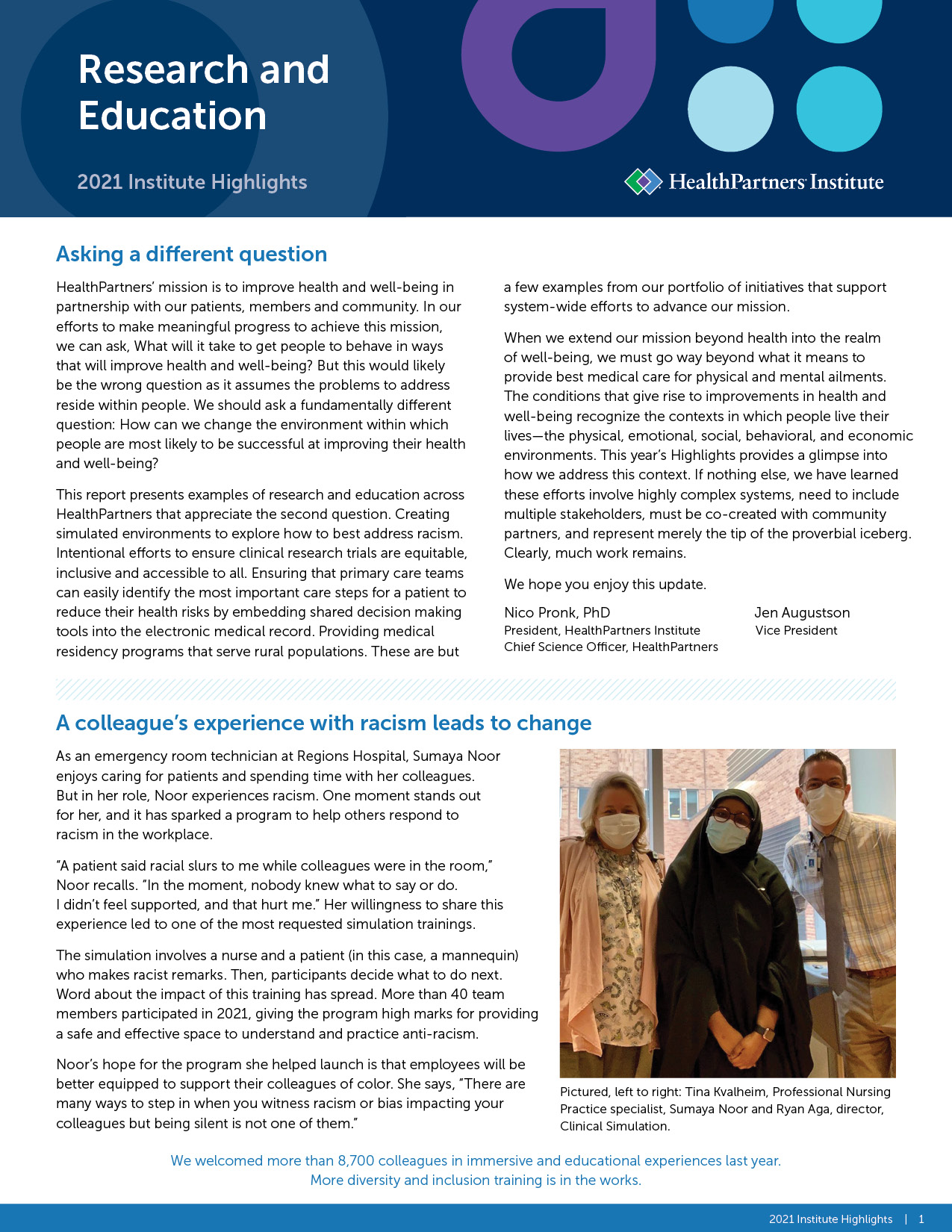**Descriptive Caption:**

The top section of the image features a blue background with various shapes, prominently displaying text in white. On the top left, it reads "Research and Education," followed by "2021 Institute Highlights." On the top right, "HealthPartners Institute" is inscribed. Below, a blue headline states, "Asking a Different Question," leading into several paragraphs of text. The opening paragraph reads: "HealthPartners' mission is to improve health and well-being in partnership with our patients, members, and community. To make meaningful progress in achieving this mission, we ask: what will it take to get people to behave in ways that will improve health and well-being?" The text is attributed to Nico Pronk, PhD, President of HealthPartners Institute and Chief Science Officer of HealthPartners, and Jen Augustine, Vice President.

In the lower section, another headline reads, "A Colleague’s Experience with Racism Leads to Change." It recounts the story of Sumaya Noor, an emergency room technician at Regions Hospital, who finds joy in caring for patients and spending time with her colleagues. Accompanying the story is a photograph on the right side, depicting three individuals wearing face masks. Sumaya Noor is in the middle, dressed in a black robe. The caption for the picture identifies the individuals from left to right as Tina Cavallin, Professional Nursing Practice Specialist, Sumaya Noor, and Ryan Agah, Director of Clinical Simulation.